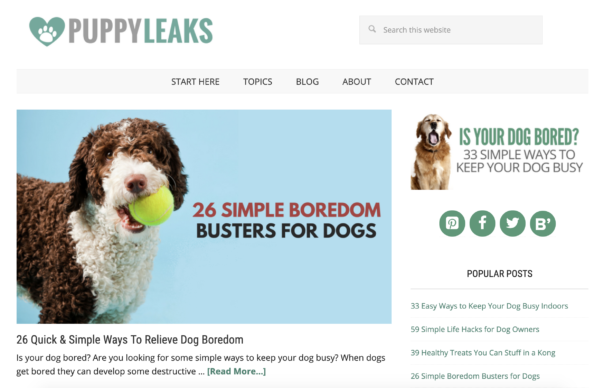This is a website layout for Puppy Leaks, displayed against a clean, white background. In the top-left corner, the website's name is prominently featured with "Puppy" in gray lettering and "Leaks" in bluish-green lettering. Adjacent to the name, there is a bluish-green heart icon with a white paw print inside. 

In the top-right corner, there is a search bar facilitating easy navigation through the site. Below this header section, a gray horizontal bar spans across the page, featuring links to different sections including Start Here, Topics, Blog, About, and Contact.

The main content is divided into two sections. On the left side, there is a clickable article. The article’s preview includes an image set against a blue background, featuring an adorable white and brown furry dog holding a yellow tennis ball in its mouth. The headline reads "26 Simple Boredom Busters for Dogs," and the subheading is "26 Quick and Simple Ways to Relieve Dog Boredom."

On the right side, another article preview is displayed, showcasing a different dog against a white background. The headline for this article asks, "Is Your Dog Bored?" and offers "33 Simple Ways to Keep Your Dog Busy."

Beneath this, there are icons linking to the site's social media platforms: Pinterest, Facebook, Twitter, and a final icon marked with a stylized letter 'B.'

At the bottom of the page, there is a section labeled "Popular Posts," providing clickable links to four of the most popular articles on the website.